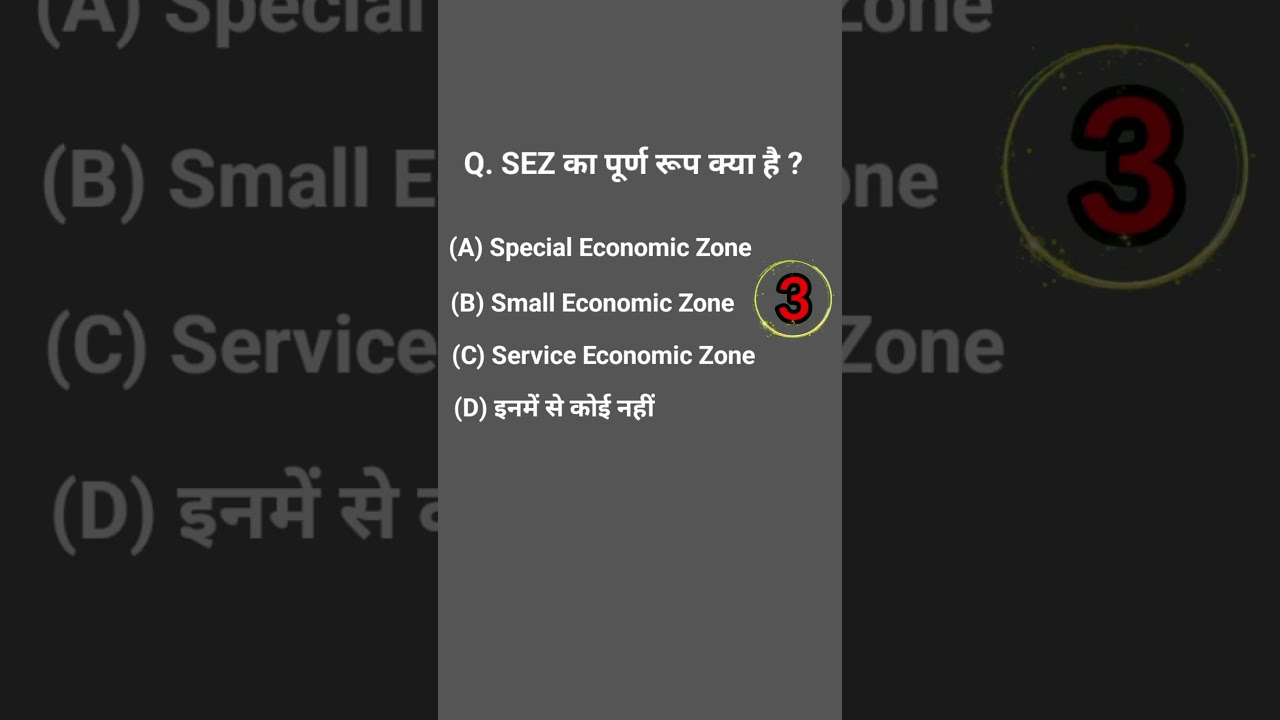This image is a screenshot from an internet source, showing a question in a quiz format over a gray background. The central part of the image features a Q followed by a question written in a language that appears to be Arabic or Indian, ending with a question mark. Below the question, there are four answer choices labeled A, B, C, and D. The answers are: A) special economic zone, B) small economic zone, C) service economic zone, and D) an option written in another language. Notably, there is a red number '3' inside a yellow circle with a black outline near the answers for B and C. On either side of the main image, there are close-ups or zoomed-in sections of the original image, grayed out, showing parts of the answer choices and the red '3' inside the yellow circle. The predominant colors in the image are black, white, gray, red, and yellow.